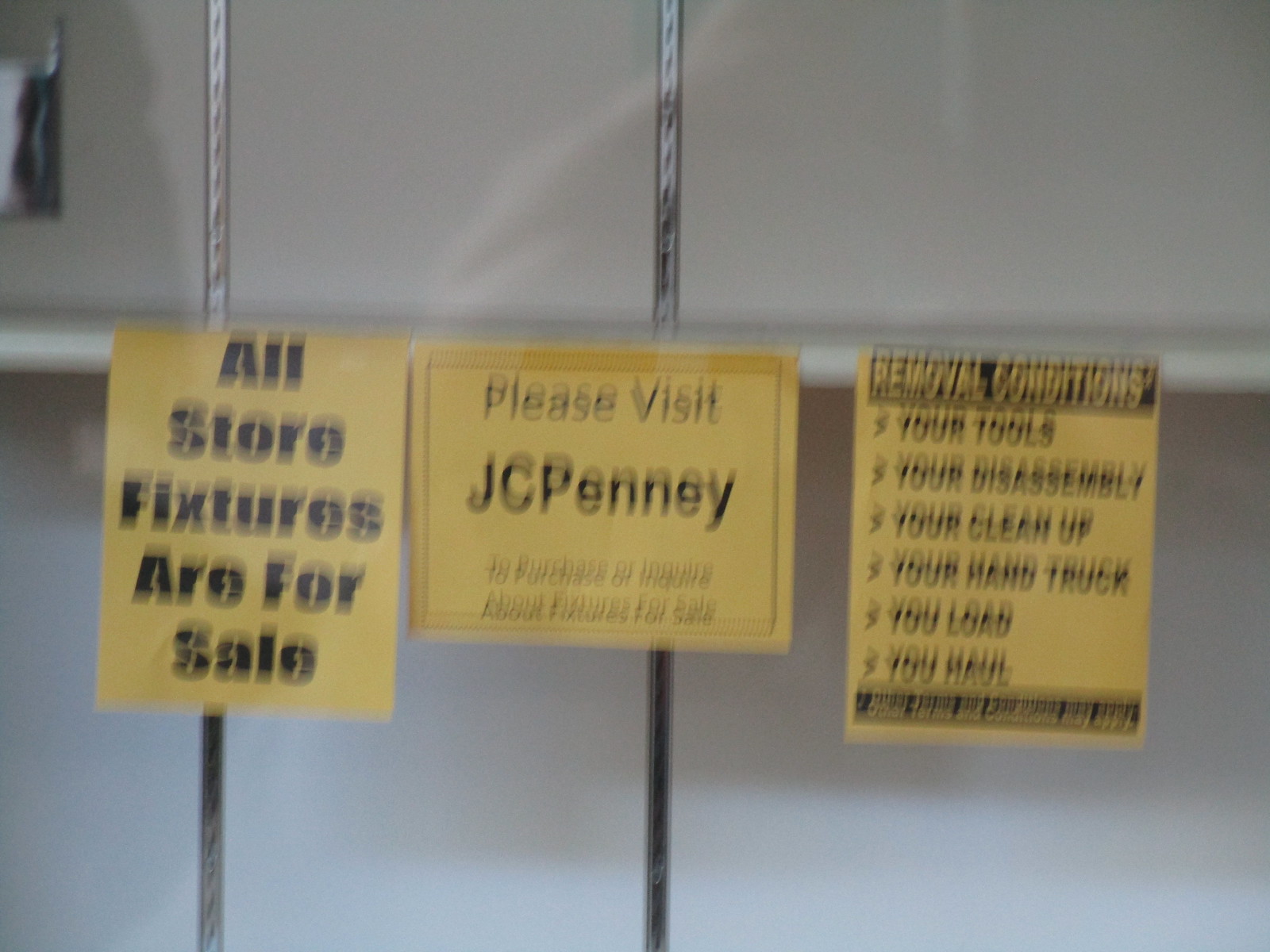Captured inside a retail store, this photograph focuses on three prominent yellow signs that convey crucial information about the store's current status. The leftmost vertical sign, with its bold black text, announces, "All store fixtures are for sale," against its stark yellow backdrop. The central, horizontally oriented sign implores shoppers, "Please visit JCPenney," and in smaller, blurrier text, it mentions something about the purchase or inquiry of fixtures, though the exact wording is difficult to discern. The rightmost vertical sign is similarly blurred, but it appears to list "Removal conditions: your tools, your disassembly, your cleanup, your hand truck, you load, you haul." All three signs are strategically placed atop empty shelving units, further emphasizing that the store is likely undergoing a closing sale, with all its fixtures up for grabs.